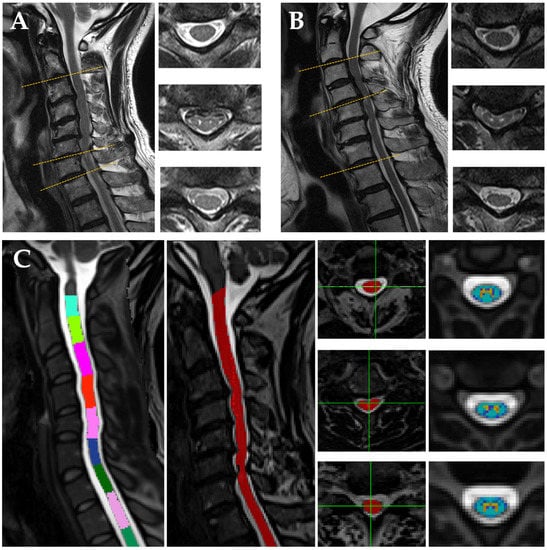The image presents a detailed medical visualization, likely an x-ray or MRI, focused on the spine. Highlighted with labels A, B, and C, the top left section (A) displays a black and white image of the spine from a lateral view, showcasing individual vertebrae or discs. To the right of this are three smaller, oval-shaped cross-sectional images of the spine, providing a top-down view of the vertebrae. Image B, positioned below, continues with similar oval cross-sections, targeting specific parts of the spine with green lines. Image C, at the bottom left, features a colorful representation of the spinal cord, with sections marked by rainbow hues including blue, green, purple, red, and pink, indicating various aspects of spinal anatomy or possibly different imaging techniques. The bottom right section includes six additional cross-sectional images, echoing the previous detailed views, and emphasizing key structural elements of the spine.